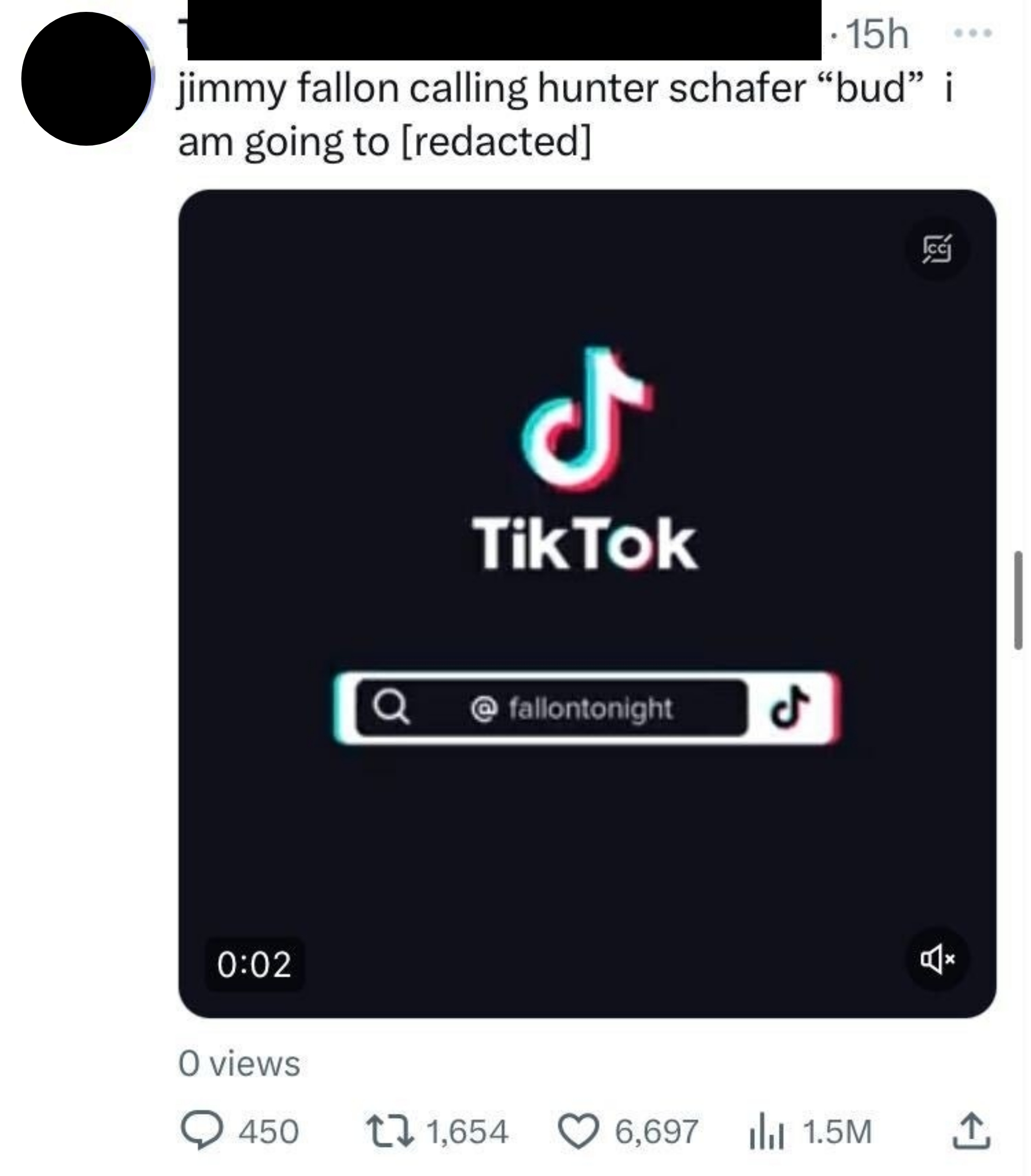### Detailed Description of the Screenshot:

This image captures a screenshot of a TikTok account, featuring an interface with several user interactions and details partially obscured for privacy. In the upper left of the screenshot, there is a circular icon that has been blacked out to conceal the user's profile picture. Additionally, the user's TikTok handle is concealed with a black bar for anonymity. 

To the right of this blacked-out area, the screen shows "15H," indicating that the post was made 15 hours ago. Adjacent to this timestamp, there are three gray dots, likely representing a menu for additional options.

Below the black bar where the user's handle is located, the text reads: "Jimmy Fallon calling Hunter Schaefer, 'bud'." Following this text, there's a statement which is partially redacted within brackets. Beneath this line, a prominent black box is displayed in the middle of the screen, featuring the word "TikTok" along with a musical note resembling the letter D.

Further down, a search bar is evident alongside a search icon and another TikTok logo. Centered on the screen, the text "@FallonTonight" denotes the user’s handle. 

At the bottom left of the image is a timestamp "0:02," signifying a short video duration, while the bottom right displays a speaker icon with an X in front, indicating the video is muted. Directly below this, "0 views" is shown alongside an icon resembling a speech bubble marked with "450 responses," tallying the number of comments.

Additionally, arrows pointing upwards and downwards denote that the post has been shared or retweeted 1,654 times. Next to this, a heart symbol indicates that the post has been liked 6,697 times. There is a series of bars—small and tall—whose specific function isn't clear but are labeled "1.5M," possibly denoting view count. Finally, a small bracket lying sideways with an upward-pointing arrow represents an upload function.